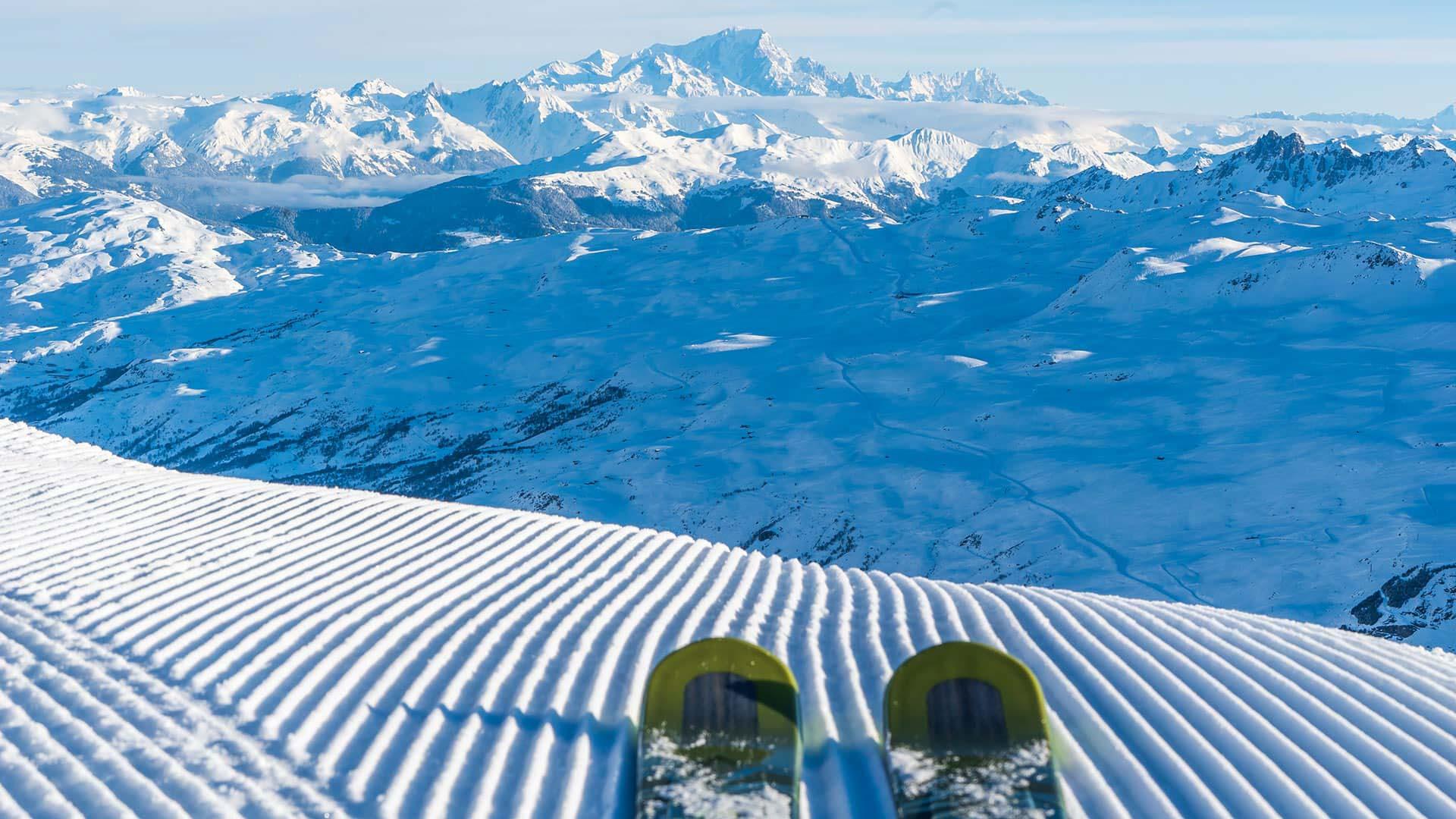At the top of a snowy slope with intricately grooved lines running downwards and towards the left, a snowboarder prepares to descend. The tips of two yellow snowboards with black interiors, dusted with snow, peek into the foreground. Below, a vast valley stretches out, covered in a thick blanket of snow, with occasional rock outcrops breaking through the white expanse. In the distance, towering, jagged mountain peaks capped with snow touch a sky that transitions from light blue to white clouds, blending almost seamlessly with the snowy landscape. This scenic view captures the serene and majestic beauty of a winter wonderland.